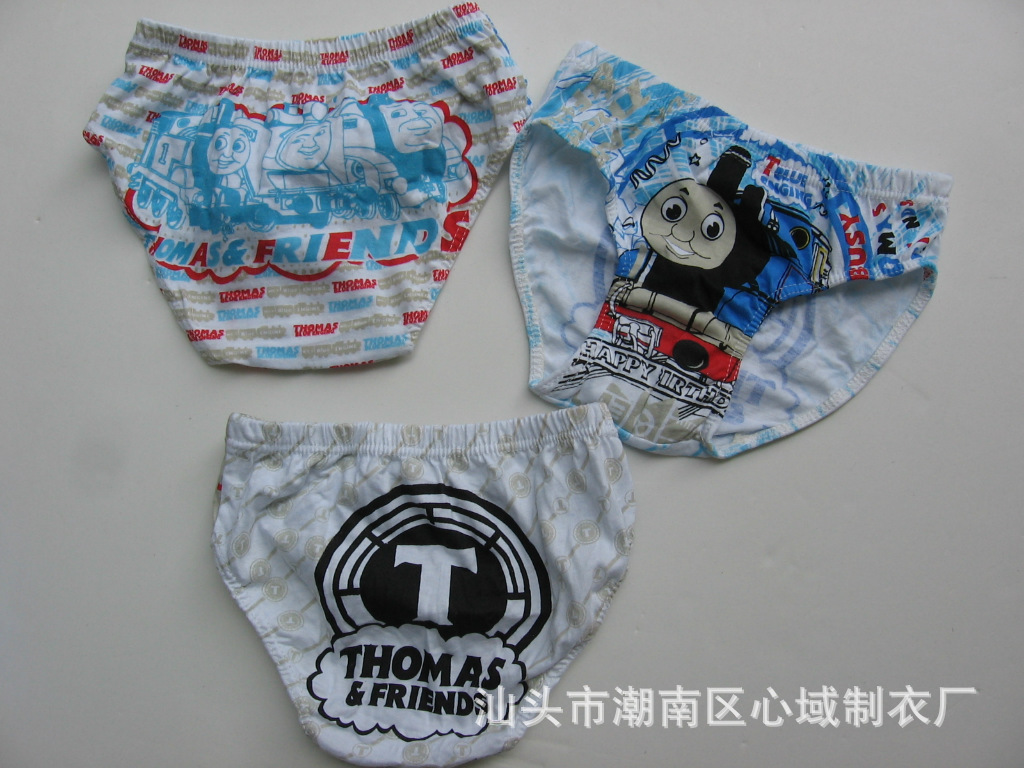The image depicts a product photo featuring three pairs of toddler underwear, all themed around Thomas and Friends. The pairs are neatly arranged on a gray or white surface. The pair on the upper left showcases three characters from the Thomas and Friends series, with blue, red, and grey accents and some text that can't be clearly discerned. The pair on the upper right displays a colorful image of Thomas the Tank Engine, smiling brightly. The pair on the bottom has a white and grey tie-dye design featuring a blue "T" and the Thomas and Friends logo in a cloud. Additionally, there is a watermark in the lower right corner of the photo that appears to be in Chinese.